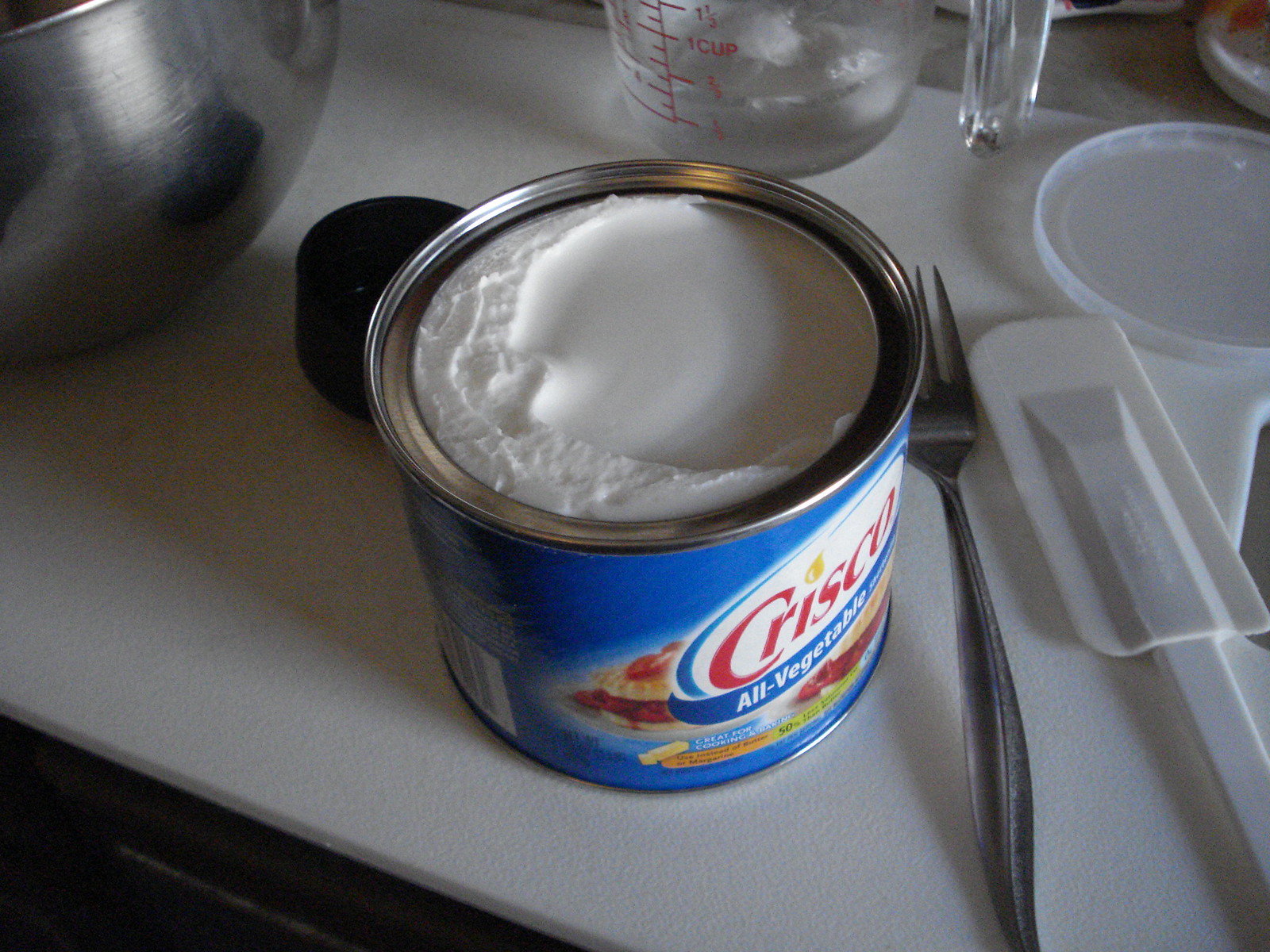This indoor photograph captures a freshly opened can of Crisco All-Vegetable Shortening, prominently displaying the blue label with red and yellow accents. The can, filled to the brim with a pristine, white, creamy substance, is placed on a white surface, likely a cutting board or countertop. Situated around the can are various kitchen tools: a silver fork, a white plastic spatula, and a two-cup glass measuring cup containing about half a cup of water and an ice cube. A steel bowl is also visible to the left, along with the plastic lid of the Crisco container. The scene suggests an immediate preparation or baking process, with the white surface enhancing the clarity of each item. The photo, taken with a personal camera, showcases these elements vividly, emphasizing the freshness and readiness of the ingredients for use.